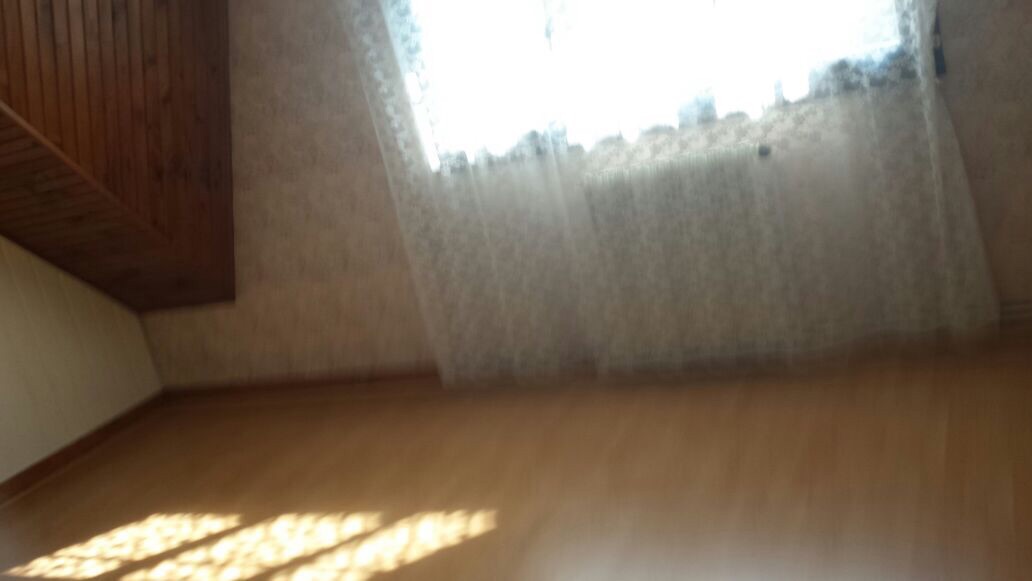The photograph, taken indoors within a residence, captures a cozy corner of a room. The room features a light brown wood floor, juxtaposed against walls adorned with creamy wallpaper. A dark brown wood-paneled accent piece occupies a corner, complemented by a matching dark brown running board at the base of the wall. Although the image is slightly blurry, the central focus is a large window allowing a flood of bright sunlight to filter through. The window, partially cropped out at the top, is covered by a delicate, translucent lace curtain in white, casting a soft, diffused glow throughout the space. This intimate scene suggests a warm and inviting domestic environment.